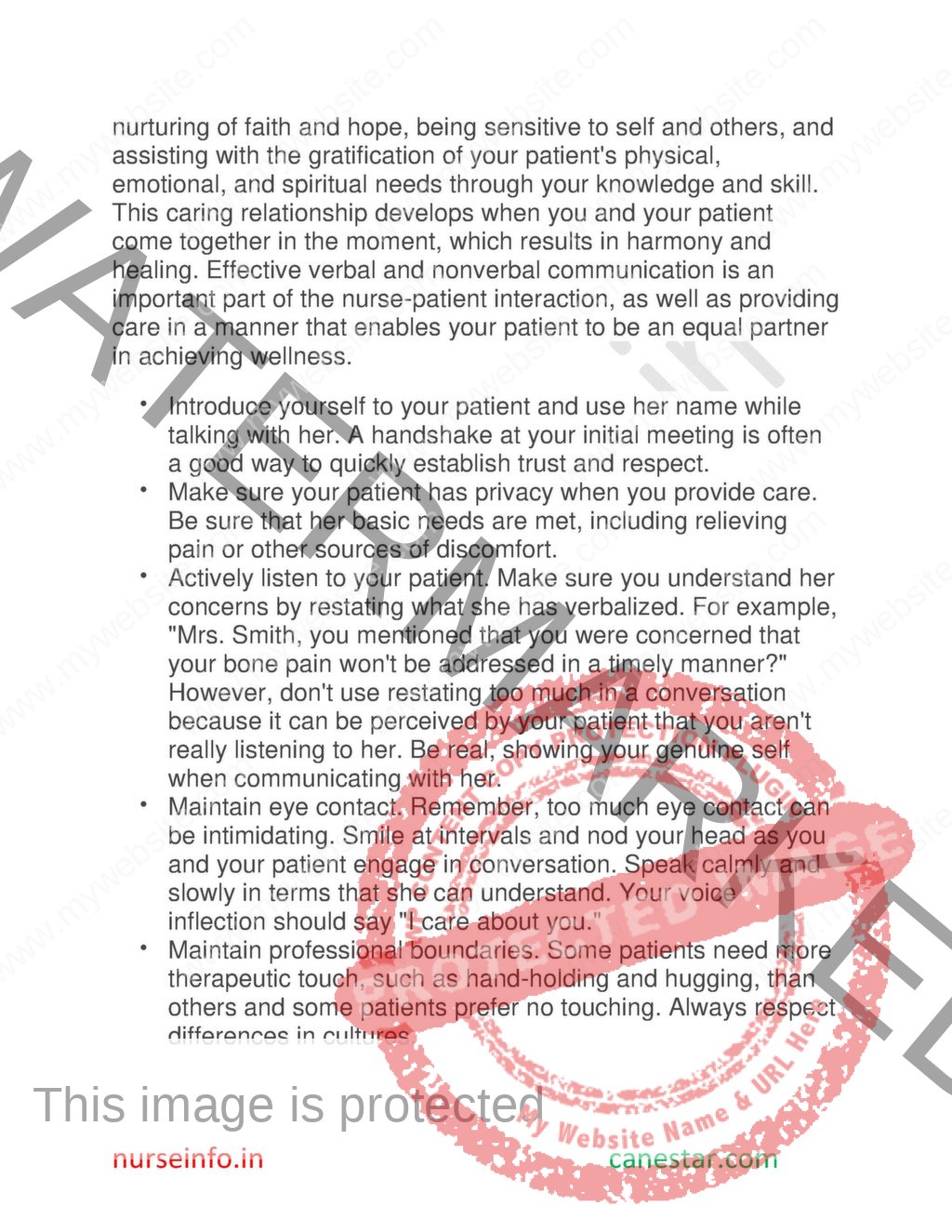The image has a white background with a diagonal black watermark that reads "WATERMARK" in capital letters. A red stamp-like graphic states "PROTECTED IMAGE." At the bottom, the text reads "This image is protected by dirt nurse info."

Behind this, in black text, is a detailed message regarding the nurturing role of a nurse: 

"Nurturing of faith and hope, being sensitive to self and others in assisting with the gratification of your patient's physical, emotional, and spiritual needs. Through your knowledge and skill, this caring relationship develops when you and your patient come together in the moment, resulting in harmony and healing. Effective verbal and nonverbal communication is an important part of the nurse-patient interaction, as well as providing care in a manner that enables your patient to be an equal partner in achieving wellness."

Below this statement, several bullet points provide practical advice for nurses:

- Introduce yourself to your patient and use her name while talking with her. A handshake at your initial meeting is often a good way to quickly establish trust and respect.
- Ensure your patient has privacy when you provide care. Be sure that her basic needs are met, including relieving pain and other sources of discomfort.
- Actively listen to your patient.